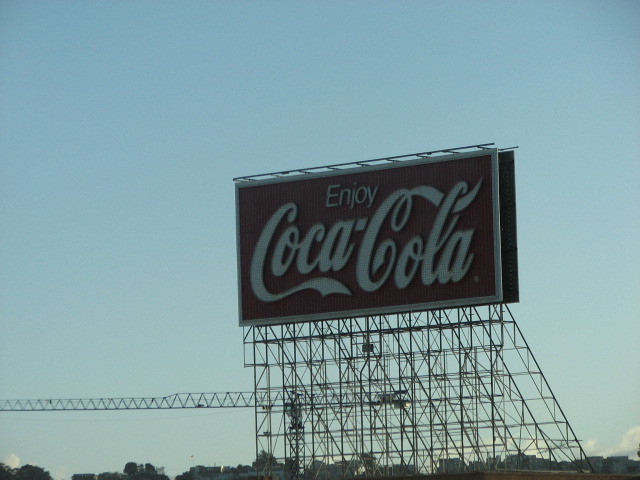The image showcases the iconic "Enjoy Coca-Cola" sign, mounted on incredibly high scaffolding. The original Coca-Cola sign, featuring its trademark white script lettering, stands out prominently, though its red background is not visible. The scaffolding structure appears see-through, suggesting maintenance or construction work, as evidenced by a crane extending from the side towards the center of the sign. To the left, additional scaffolding ascends vertically. The impressive height of the structure is emphasized by the small appearance of the buildings below and the cloud line, which hovers above the buildings but well below the Coca-Cola sign. The scene is set against a clear blue sky, with no other elements visible in the background.